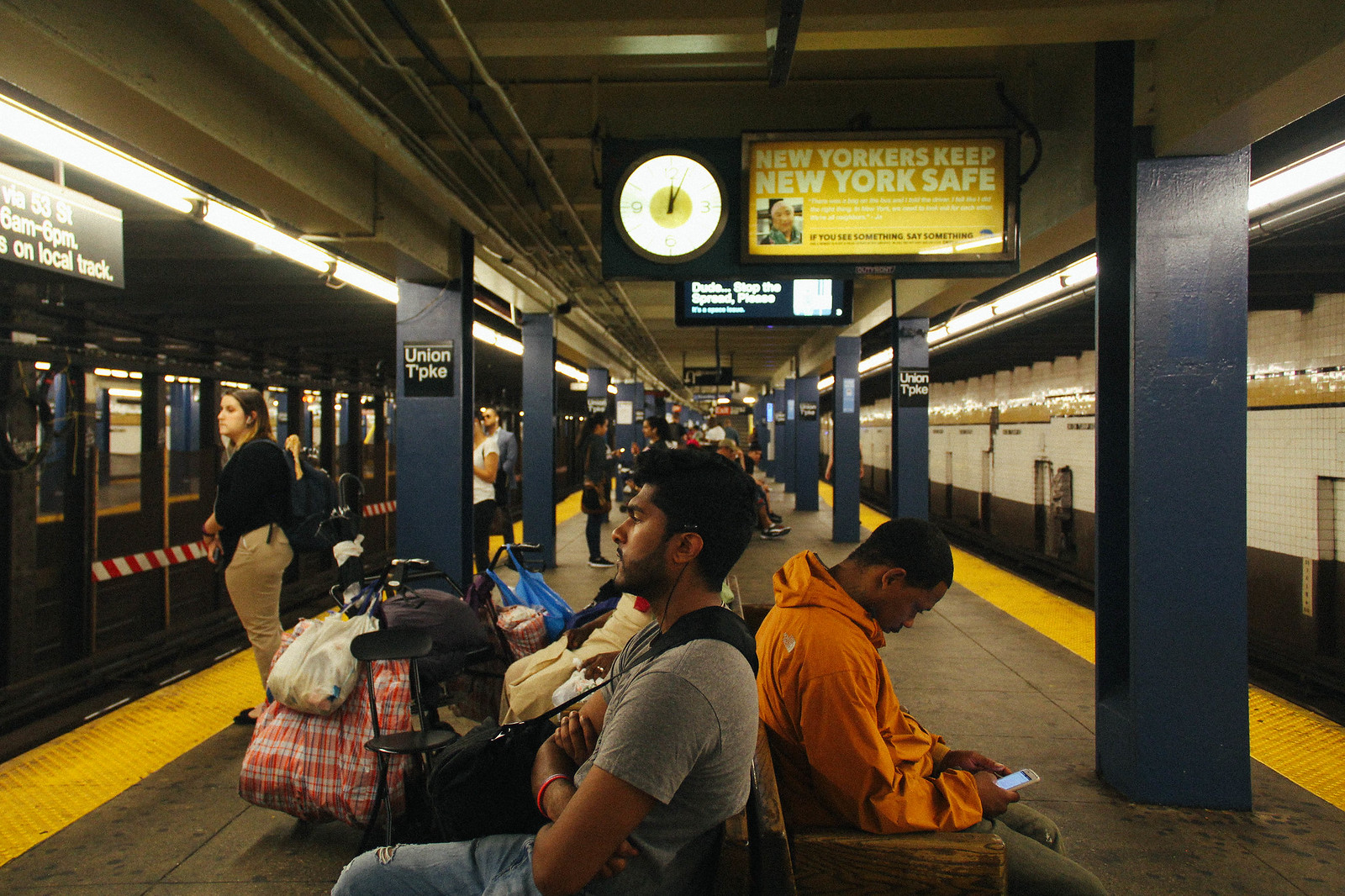This detailed image captures the bustling interior of a New York City subway station. At the top of the photo, a yellow sign with white print prominently displays the message, "New Yorkers Keep New York Safe," situated beside a clock with a black background and white hands, showing the time as a little after 12. The station platform is lined with a diverse array of passengers, both seated and standing, awaiting their trains. 

In the forefront, a man in a gray t-shirt and blue jeans sits with his arms folded across his chest, staring straight ahead at a subway car that has just arrived on the left side of the frame. To his right, a gentleman in an orange hoodie is engrossed in his phone. Behind them, more people sit on benches and stand near the platform edge, where a yellow safety line separates them from the tracks.

The left side of the image features a stationary subway train with its doors open and passengers poised to board. On the right side, there is no train, revealing a white and brown concrete wall across the tracks. Blue columns labeled "Union Turnpike" recede into the background, emphasizing the depth of the terminal. Scattered belongings, including bags and a chair, sit next to the man in the gray shirt, adding to the lived-in feel of the scene. The atmosphere is typical of a New York subway: crowded, diverse, and alive with the constant flow of city life.